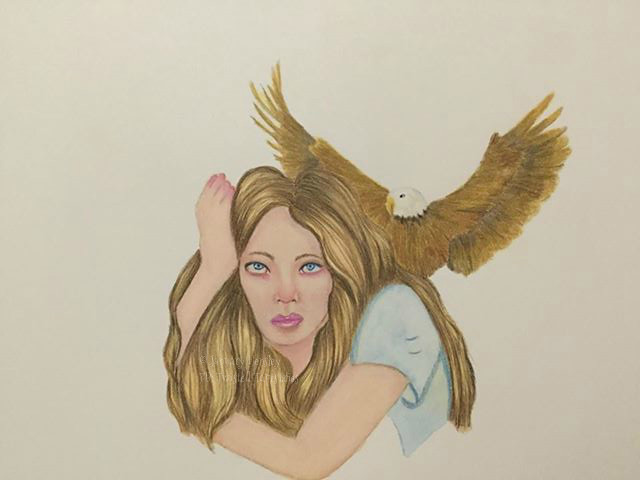This detailed sketch depicts a sorrowful woman with blue eyes and dirty brown hair accented by blonde highlights. Her right hand rests pensively on her temple, while her left arm is folded, presumably leaning on an unseen surface. Her left hand is obscured by her cascading hair, which flows down her back. She is clad in a blue short-sleeved shirt. 

An eagle, colored similarly to her hair, with a white head and brown beak, is prominently featured beside her. The eagle also has a slightly darker brown collar. Despite the gray background, the woman's delicate features stand out, accentuated by her pink lipstick and the pinkish hue beneath her eyes. Her gaze is cast upwards, amplifying the profound sadness that emanates from her expression.